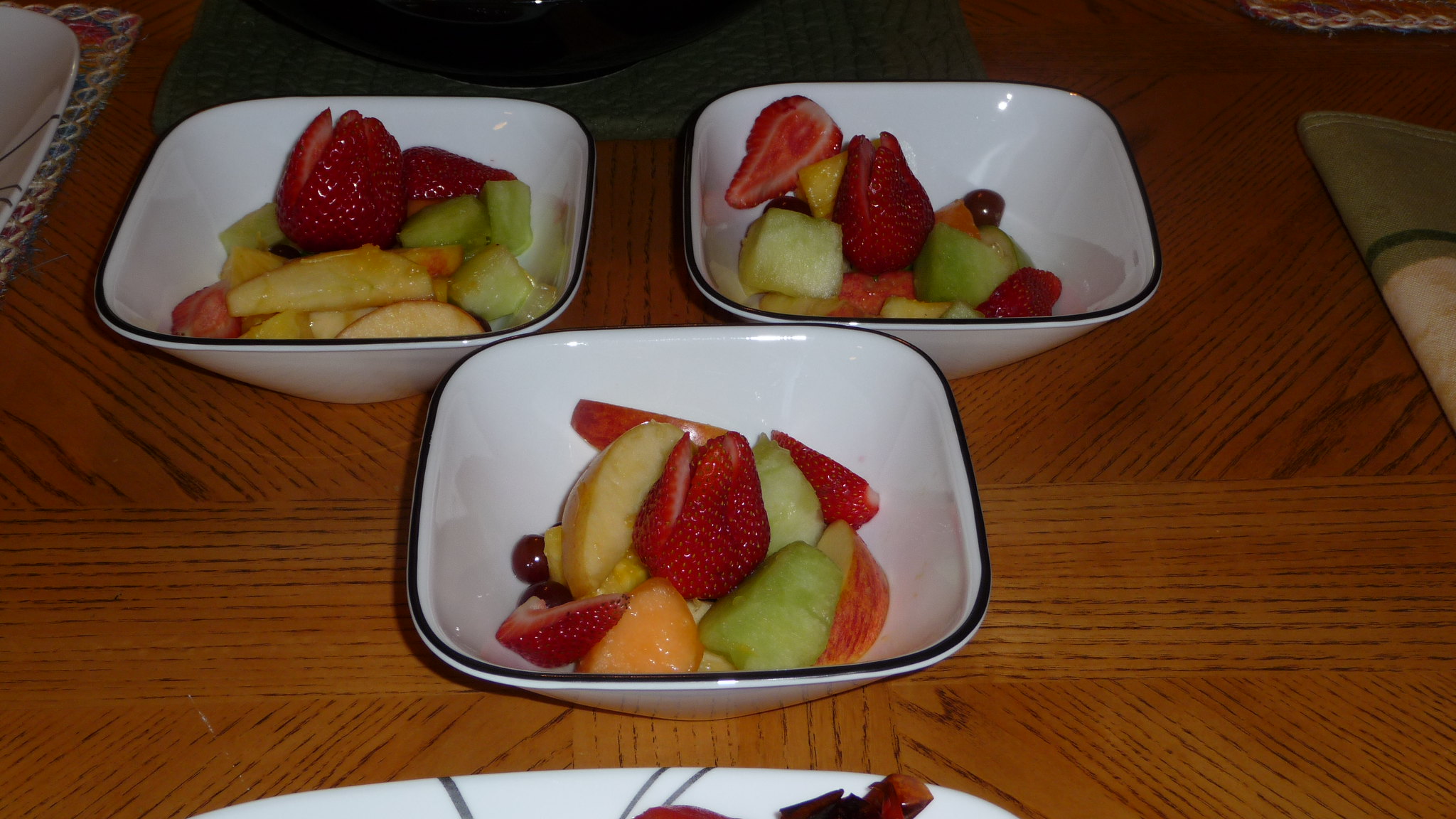This photograph features a brown wooden table with three white, square bowls adorned with black edges, meticulously arranged to resemble two eyes and a nose—two bowls at the top and one centered beneath them. Each bowl holds a colorful fruit salad, showcasing slices of strawberries, honeydew, apple, cantaloupe, and clusters of red grapes. To the right is a green and tan cloth napkin, adding a touch of rustic elegance to the scene. The table also includes partial glimpses of two other plates: one peeking from the bottom of the image and another subtly framed in the bottom-right corner. The table itself has a distinguished appearance, marked by its long, striped edges. This comprehensive arrangement invites viewers into a harmonious blend of colors and textures, perfectly capturing a moment of simple culinary delight.